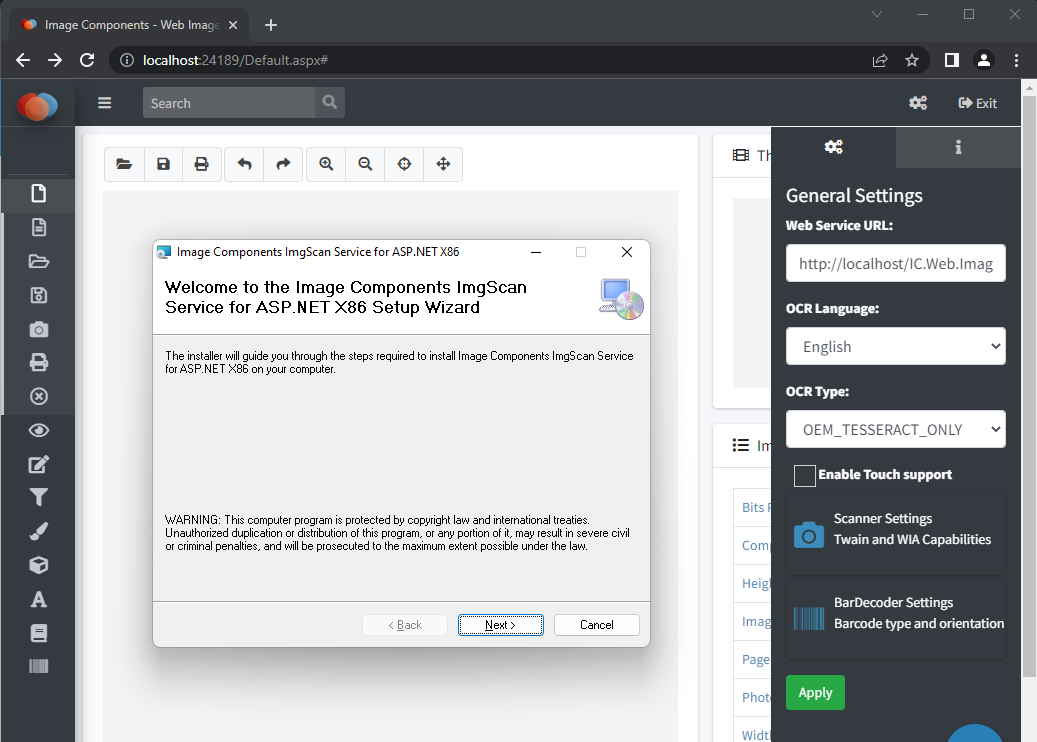This is a detailed screen capture of a website displayed on a computer screen or tablet in landscape mode. The website interface predominantly features white and gray colors with subtle accents of additional shades such as blue, green, and a branded logo in the upper left corner. The logo comprises three overlapping egg-shaped circles in red, orange, and light blue, ordered from left to right.

The left side of the screen hosts a vertical stack of navigation icons, which seem to be related to image editing functionalities. The top of the webpage prominently displays the heading "Image Components Web Images," and directly beneath this is the URL, "localhost:24189/default.aspx," followed by a hashtag, indicating a local server environment.

The browser window operates in night mode, with the browser's frame and any pop-ups being dark gray. In the central section of the webpage, the background shifts to lighter gray and white hues. A pop-up window dominates this area, presenting the message: "Welcome to the Image Components Image Scan Service for ASP.NET x86 Setup Wizard," accompanied by navigation buttons labeled "Back," "Next," and "Cancel."

On the right side of the screen, there is an additional menu dedicated to general settings, contributing to a user-friendly layout designed to facilitate ease of navigation and functionality.